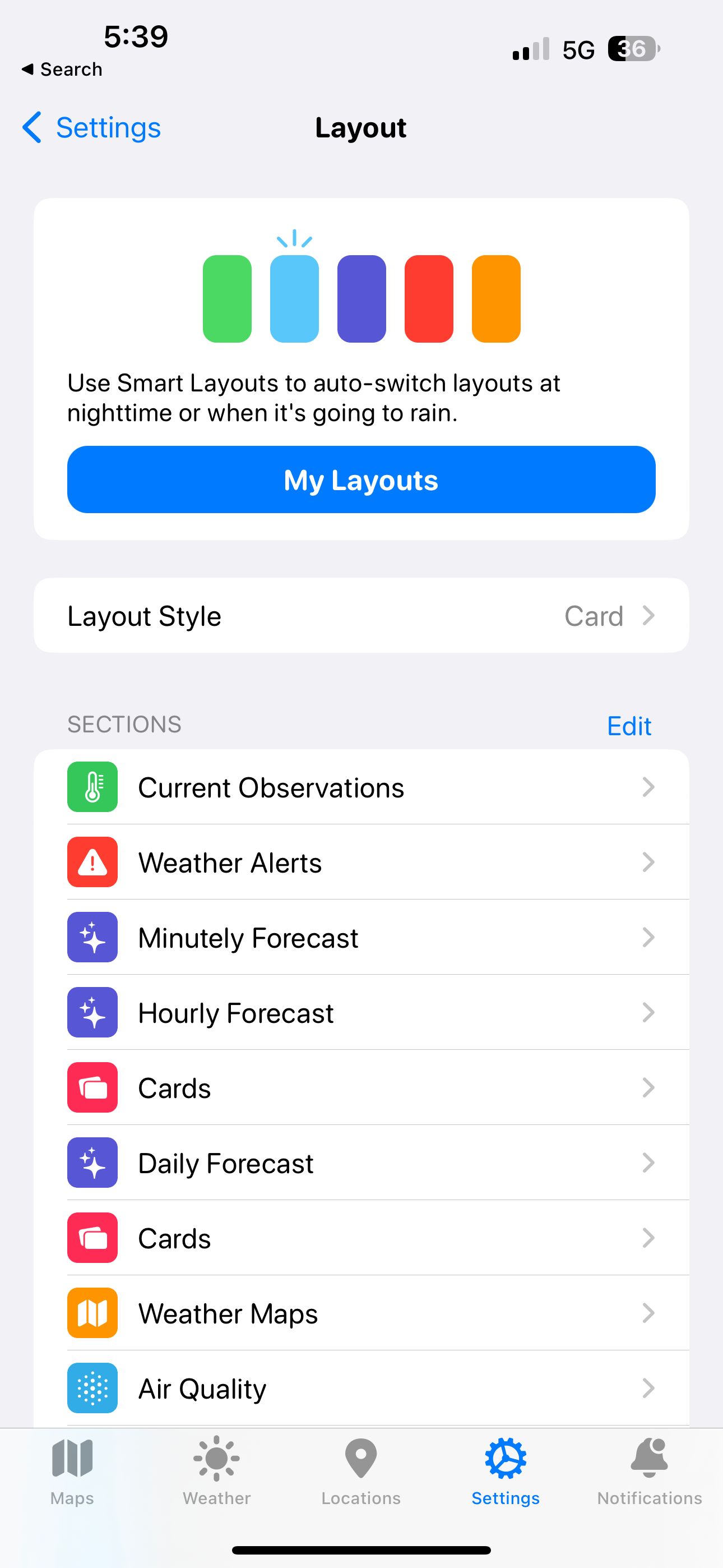The image is a detailed screenshot of an iPhone at 5:39 AM, judging by the digital time displayed in the top left corner. The phone shows a 36% battery level, alongside a 5G indicator and a two-bar signal strength icon. Below the time, the screen displays a search bar with a left-pointing black arrow next to it. Directly below the search bar is the word "Settings" in a prominent blue text, accompanied by another left-pointing arrow. 

Centrally aligned at the top, the screen highlights the "Settings" header, with a black-colored layout button to its right. Beneath this, there is a distinctive boxed section containing five vertical rectangles sequentially colored green, blue, purple, red, and orange. Below this colorful column, the box is labeled "My Layouts" in white text set against a blue background.

Moving further down, the screen indicates a segment titled "Layout Style" with the word "Card" next to it. The bottom half of the image showcases a list of various section names grouped under the overarching title "Sections." The orderly layout and use of vibrant colors suggest it might be part of a design or customization app, reflecting a structured user interface configuration.